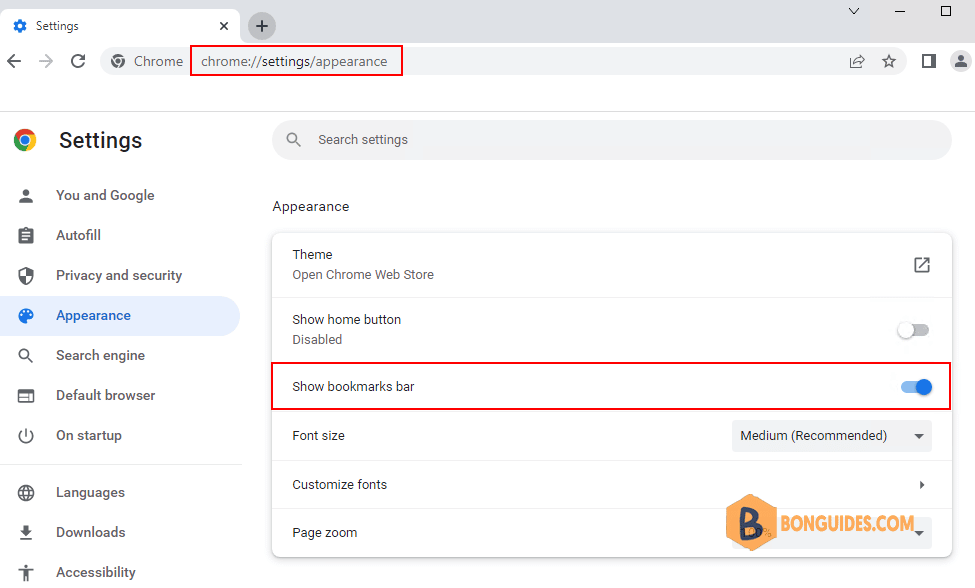The image depicts a computer screen displaying the Google Chrome settings page, specifically the "Appearance" section, accessed via the URL "chrome://settings/appearance." The browser window shows only one tab open, which features a blue gear icon labeled "Settings." The main content area of the screen is highlighted with a red rectangle, focusing attention on a particular section within the settings.

At the center of the screen, another red rectangle encompasses a specific setting labeled "Show bookmarks bar." This section features a white background and a blue slider, currently switched to the "On" position, indicating that the bookmarks bar is enabled.

On the left side of the screen, there is a vertical menu consisting of several icons with corresponding labels. These labels include "You and Google," "Autofill," "Privacy and security," "Appearance," and "Search engine," among others, extending down the side of the settings menu. The top of this menu displays the Google Chrome icon, emphasizing the browser being used. The overall background of the settings page is gray, providing a neutral backdrop for the highlighted content.